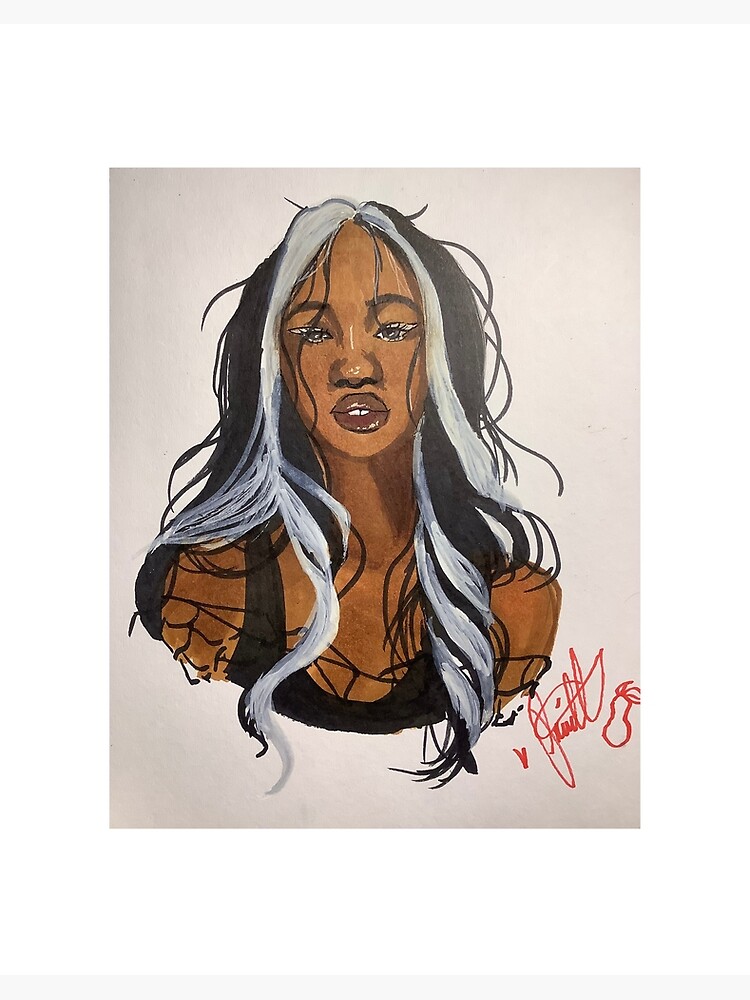This is a detailed portrait of a young woman of either African or mixed Asian descent with distinct two-tone hair, primarily black with white streaks and highlights, and curly sections at the front. Rendered in a casual, loose style that might be colored marker or watercolor, the portrait captures her head, shoulders, and upper torso against an off-white, blank background, with the rest of her body gradually fading into it. She has dark grayish eyes with heavy mascara, wears white eyeliner, dark burgundy lip gloss, and a black tank top. Her expression is neutral, with her mouth slightly parted, revealing her teeth. The artist's mostly unreadable cursive signature appears in red ink at the bottom right, along with a small drawing resembling a gourd with hair.